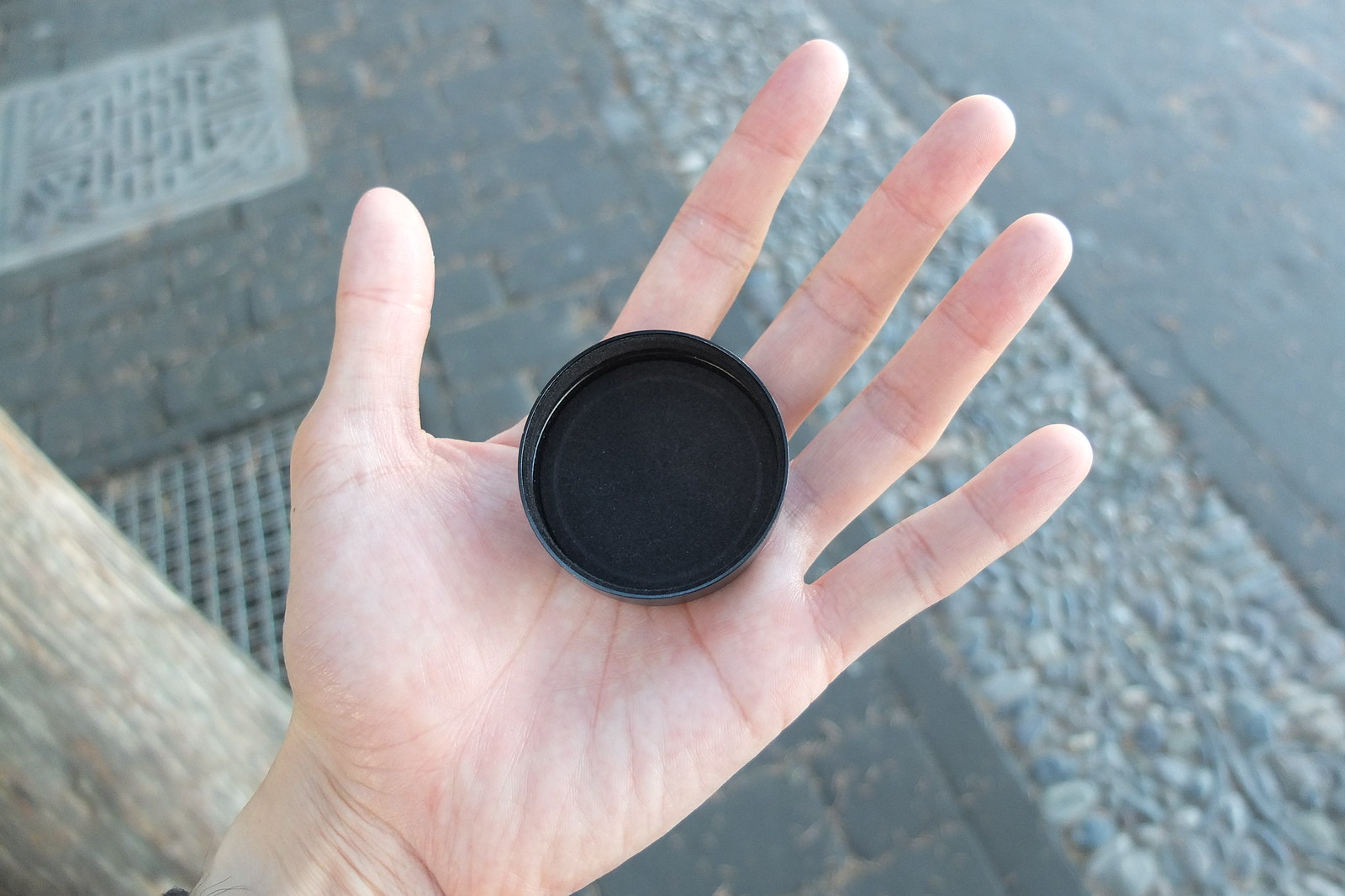This photograph captures a pale left hand with the palm facing upwards, outstretched fingers and thumb, and holding a pitch-black circular cap or lid, which may be a camera lens cap. The black cap is small and centered in the hand. Taken outside, the image orientation shows the hand pointing slightly upward and to the right. The background features dark gray cobblestones and two grates embedded in the ground; one grate is dark gray, blending with the stones, while the other stands out in a lighter gray shade. In the lower left corner, there is a light gray-brown wooden object, possibly a tree trunk or a post. Visible lines of stones run diagonally toward the right of the photo, adding texture and depth to the scene.